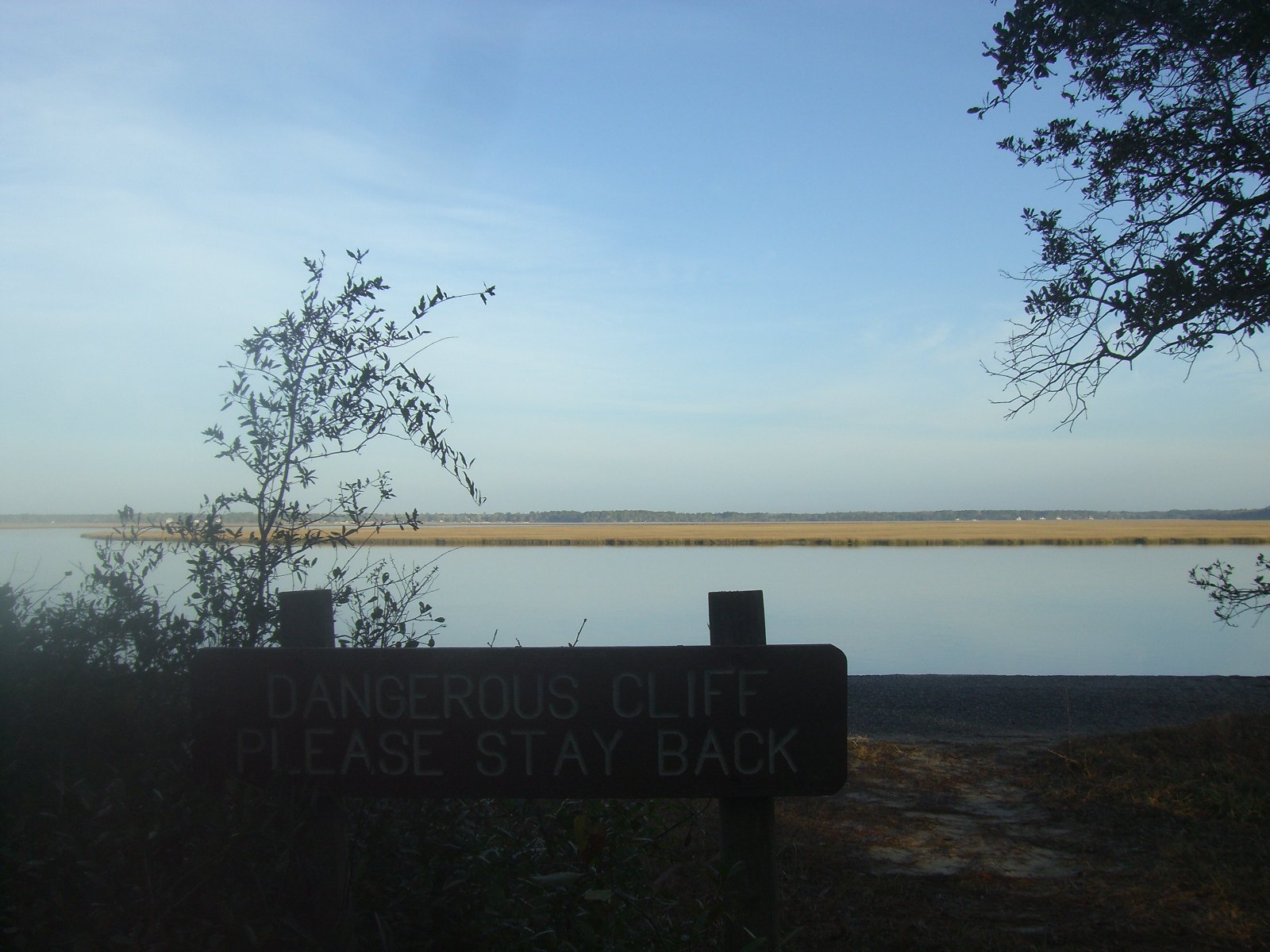The image captures a serene yet cautionary scene of a lake or pond bordered by a potentially hazardous cliff. At the base of the cliff, a rectangular wooden sign, supported by two wooden posts, is prominently displayed, warning with the words: "Dangerous Cliff. Please Stay Back." Flanking the sign, clusters of trees are visible on both the left and right sides, enhancing the natural ambiance of the area. A wooden path weaves through the landscape, adding a rustic charm to the location.

In the backdrop, there's a vast, orangish field leading up to a distant range of mountains, suggesting an expansive and open terrain. The scene is set against a sky that, though partly cloudy, indicates the brightness of early morning or perhaps evening, casting a warm glow on the surroundings. Over to the far side of the lake, one can faintly discern the shape of a city, adding an element of human presence to this otherwise natural setting. The image encapsulates a tranquil yet slightly perilous beauty of nature, inviting caution as well as admiration.